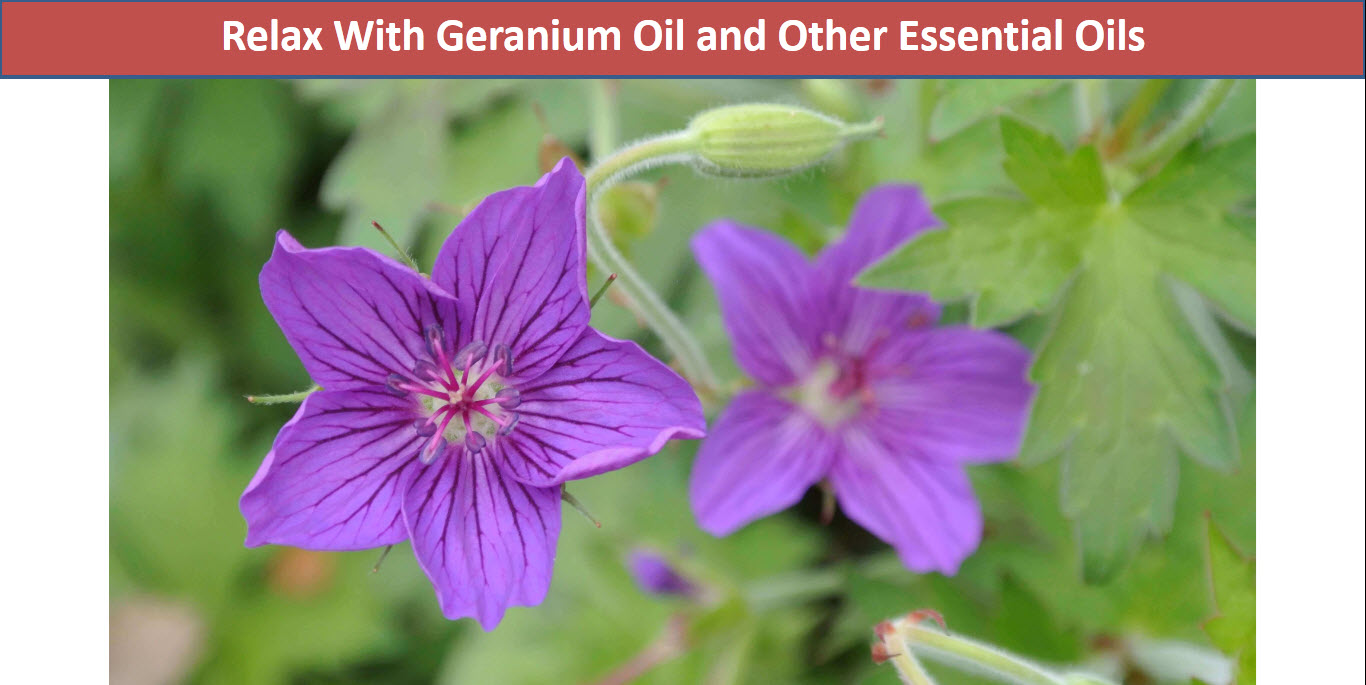The close-up photo captures the serene beauty of two large geranium flowers, their petals a lighter purple adorned with intricate, darker purple veins and centers that bloom brightly. Nestled amongst them is a budding geranium, with a backdrop of vibrant green foliage under the clear daytime sky. Prominently displayed towards the top middle of the image is a rusted red text bar featuring bold white text that reads, "Relax with geranium oil and other essential oils." The composition suggests an advertisement for herbal remedies, inviting viewers to find calm and relaxation through the natural allure of geraniums, devoid of any human presence or additional text.